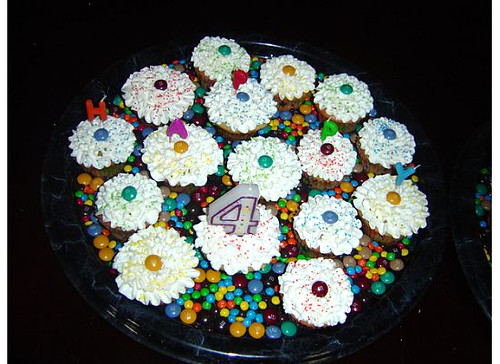This close-up photograph showcases a festive arrangement of around 16 cupcakes on a glass platter, set on a black table. The cupcakes are meticulously decorated with white icing, emulating the appearance of delicate white flowers, with each "flower" centered by a colorful M&M in various hues such as green, blue, orange, yellow, and red. Scattered around the base of the cupcakes are brightly-colored M&Ms and smaller confectionery chocolates in shades like lime green, blue, orange, yellow, maroon, dark blue, and cyan blue, creating a vibrant, playful backdrop.

Each cupcake is topped with additional sprinkles in an array of colors, adding to the delightful, whimsical presentation. This display is clearly crafted for a child's birthday celebration, evidenced by the “happy” spelled out in different colored candles (red, purple, green, and blue) and a prominent purple-outlined number four candle standing tall on a cupcake towards the bottom center. This cheerful assortment of sweets vividly marks a joyful fourth-birthday party.